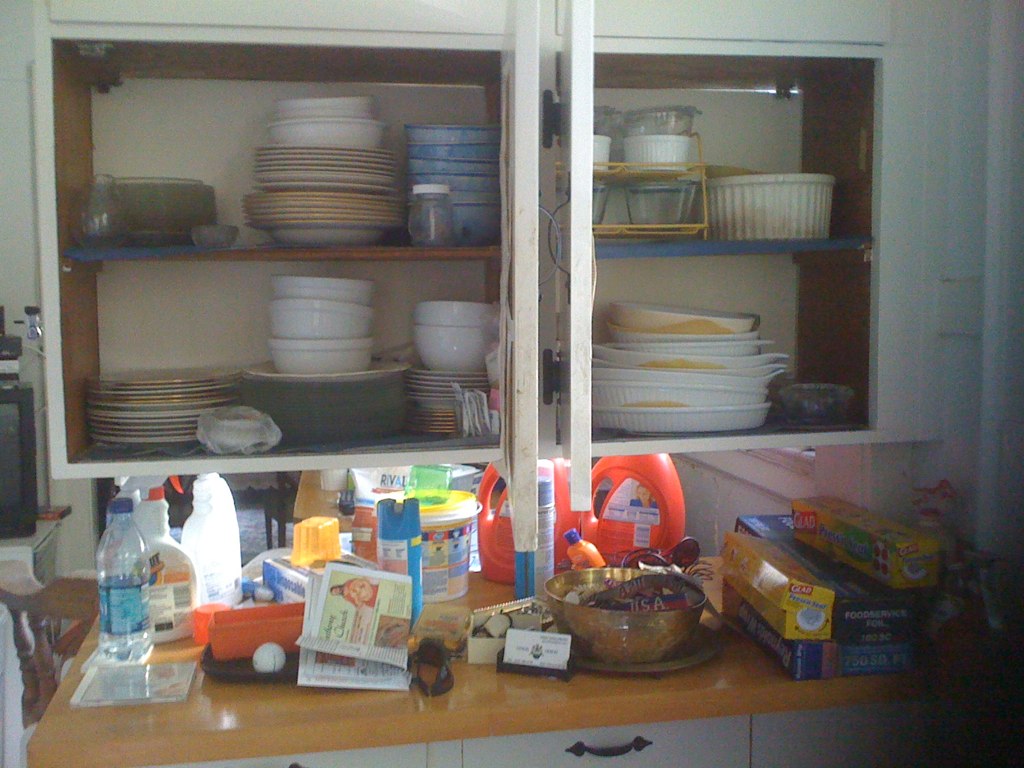This color photograph is taken within a cozy kitchen setting, featuring a small wood grain countertop paired with small white cabinets below. The cabinets appear to have three drawers, each adorned with sleek black handles. The countertop is bustling with various items. On the right side, multiple packages of GLAD brand products are neatly arranged, including rolls of tin foil, wax paper, and saran wrap, showcasing their distinct yellow, green, and metallic blue colors.

Further to the left, a yellow bottle containing washing machine soap stands prominently. In front of this bottle lies a decorative gold bowl, resting on a matching gold plate, and filled with several small packages. Nearby, a black holder securely keeps an assortment of business cards. 

The far left side of the countertop hosts a water container and a spray bottle, adding to the functional aspect of the space. Above the countertop, two white cabinets with glass doors offer a peek inside, revealing neatly stacked plates, bowls, and an assortment of clear glass containers, all attentively organized. The photograph captures a harmonious blend of practicality and aesthetic appeal in this well-utilized kitchen corner.